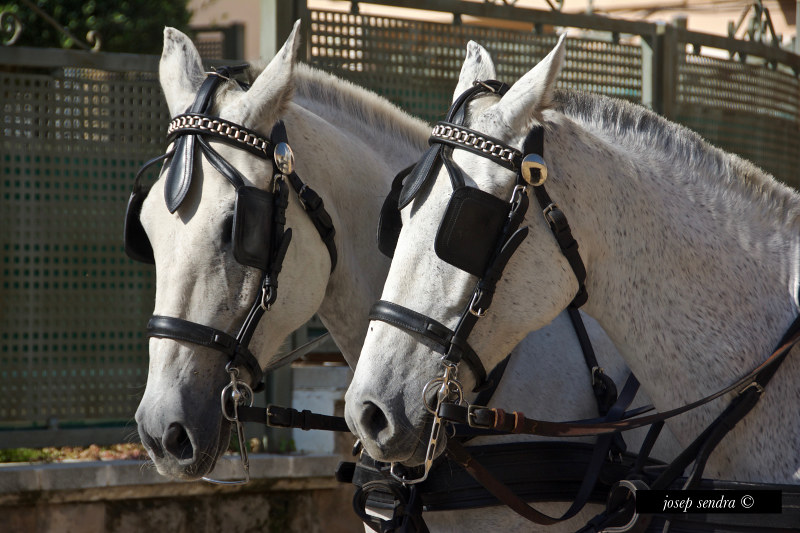This captivating photograph showcases two white horses with specks of gray, presented in a close-up side-by-side profile, looking toward the lower left-hand corner. Each horse wears black leather harnesses intricately designed with straps and square eye visors, known as blinders, which limit their peripheral vision to what is directly in front of them. Their bridles feature a decorative metal chain link across their heads, adding an elegant touch to their gear. The image suggests the horses are part of a horse-drawn carriage setup, though the carriage itself is not visible. Despite the harnesses, their short, well-groomed manes and overall appearance indicate they are well-cared for. The background reveals a patterned gray fence with horizontal rows of small open squares, adding to the serene setting. At the bottom of the photograph, a watermark in a black rectangular box displays the photographer's name, "Joseph Sandra," in lowercase white font.